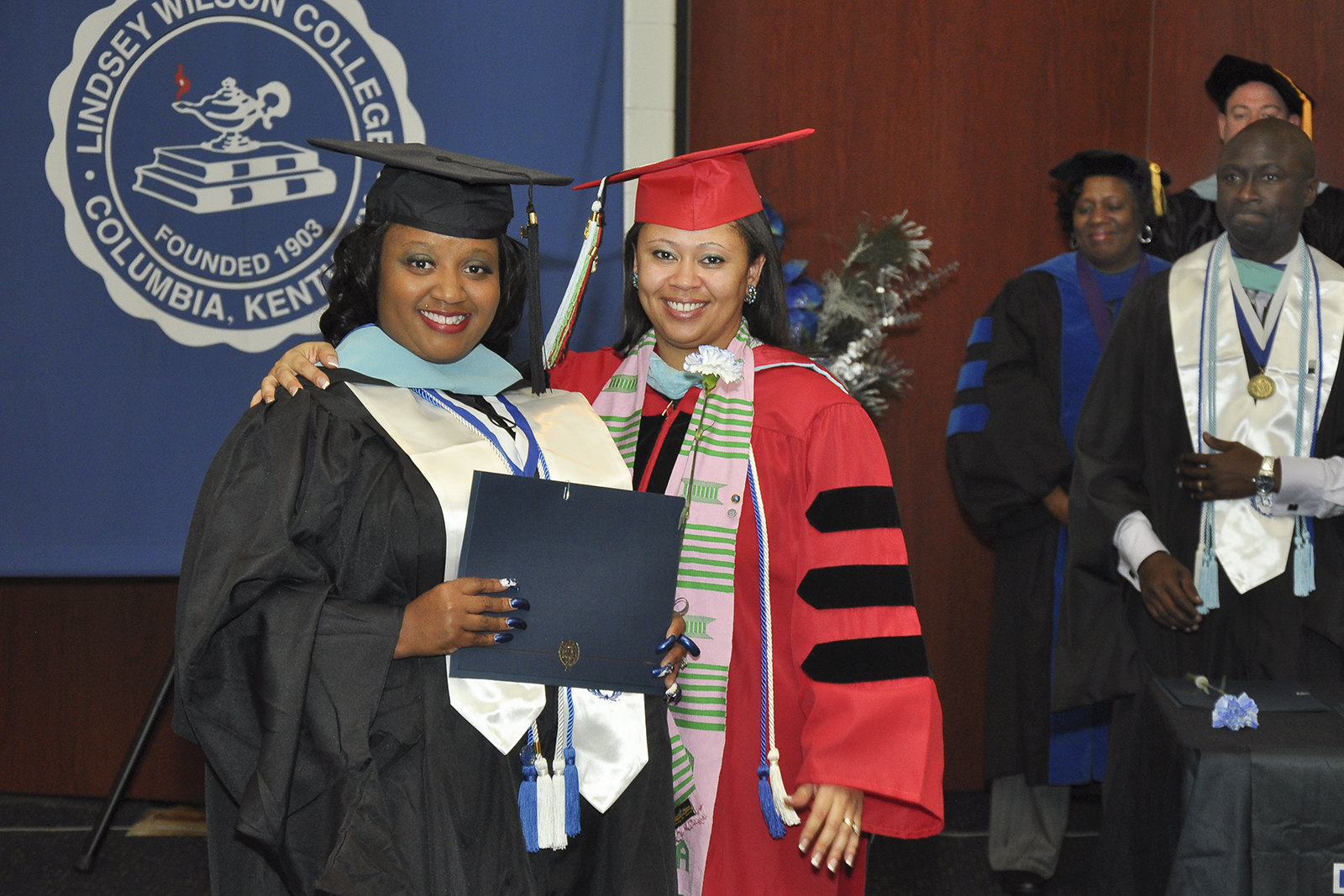The photograph captures a vibrant and joyful scene at a college graduation ceremony, likely at Lindsay Wilson College in Columbia, Kentucky, as a prominent blue banner in the background suggests. The banner, adorned with the college's name and founding year, 1903, also features the school's logo: a stack of books topped with an old-fashioned lamp emitting a red flame.

Centered in the image, two black women stand proudly. The woman on the left wears a traditional black graduation cap with the tassel on the right, a black gown, and various drapings around her neck. She is beaming with pride while holding what appears to be her diploma. Beside her, a woman dressed in a red graduation cap and gown has her arm affectionately around the other graduate, possibly conveying a mentor-student relationship. Both women display a sense of achievement and camaraderie.

In the background, three other individuals, including an older black woman in a black cap and gown and a white man in similar regalia, add depth to the scene, suggesting they too are participants in the graduation ceremony, awaiting or having just received their degrees. The overall atmosphere is celebratory, filled with the anticipation and joy that accompanies such significant academic milestones.